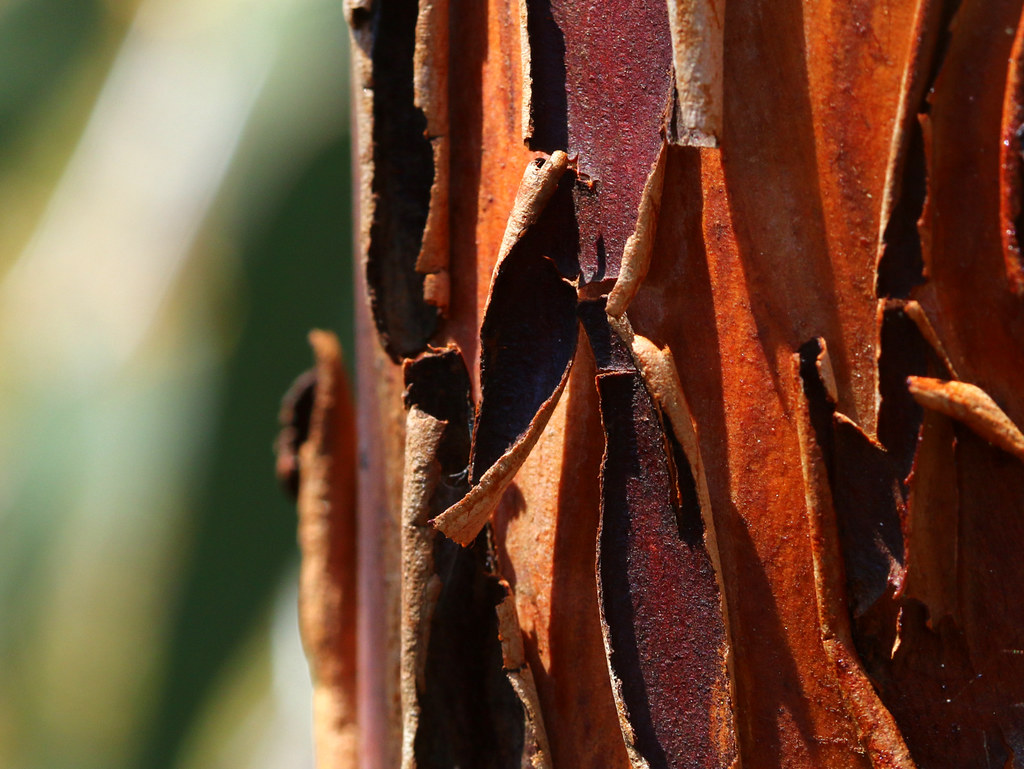The image displays a close-up, horizontally oriented shot of peeling tree bark, occupying most of the right two-thirds of the frame. The bark is dark red on the outside and curls up in strips, revealing a light brown inner surface. Beneath the peeling bark, there's an orangish-brown layer, suggesting an interesting interplay of colors. The left third of the image features a blurred background composed of mixed hues of dark green, light green, and light yellow-white, indicating a natural setting with abundant greenery and bright light. The overall impression is of an aged, textured tree trunk with vividly contrasting colors.